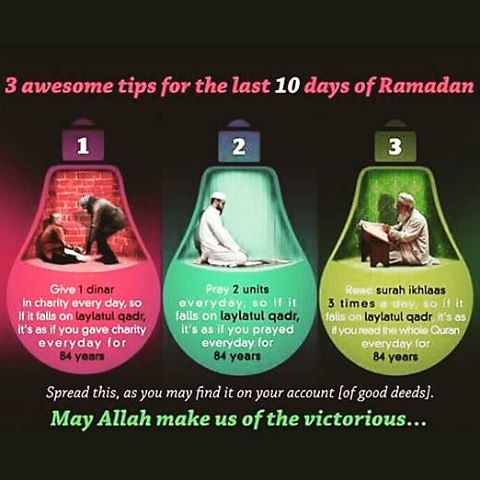The poster, designed with a solid black background, presents three actionable tips for the last 10 days of Ramadan. At the top, the text "Three Awesome Tips for the Last 10 Days of Ramadan" is prominently displayed, with "10" notably highlighted in white against the pink-colored rest of the text. The central focus is on three cartoon-styled, inverted light bulbs, representing the tips. 

The first bulb, pink and marked with the number one, features an image of two people conversing. Its accompanying text advocates giving one dinar in charity every day, emphasizing that if it coincides with Laylatul Qadar, it would equate to giving charity daily for 84 years. The second bulb is green, numbered two, with an illustration of a man praying. This tip suggests praying two units daily, highlighting that doing so on Laylatul Qadar is akin to praying daily for 84 years. The third bulb, which is yellow and numbered three, depicts an elderly man reading a book. The advice here is to read Surah Ikhlas three times a day, suggesting that if performed on Laylatul Qadar, it equates to reading the entire Quran every day for 84 years.

Below these tips, there's a motivational message encouraging viewers to "Spread this as you may find it on your account of good deeds," written in white text. The concluding line, in green text, reads, "May Allah make us of the victorious," offering a prayerful wish for success and blessings.